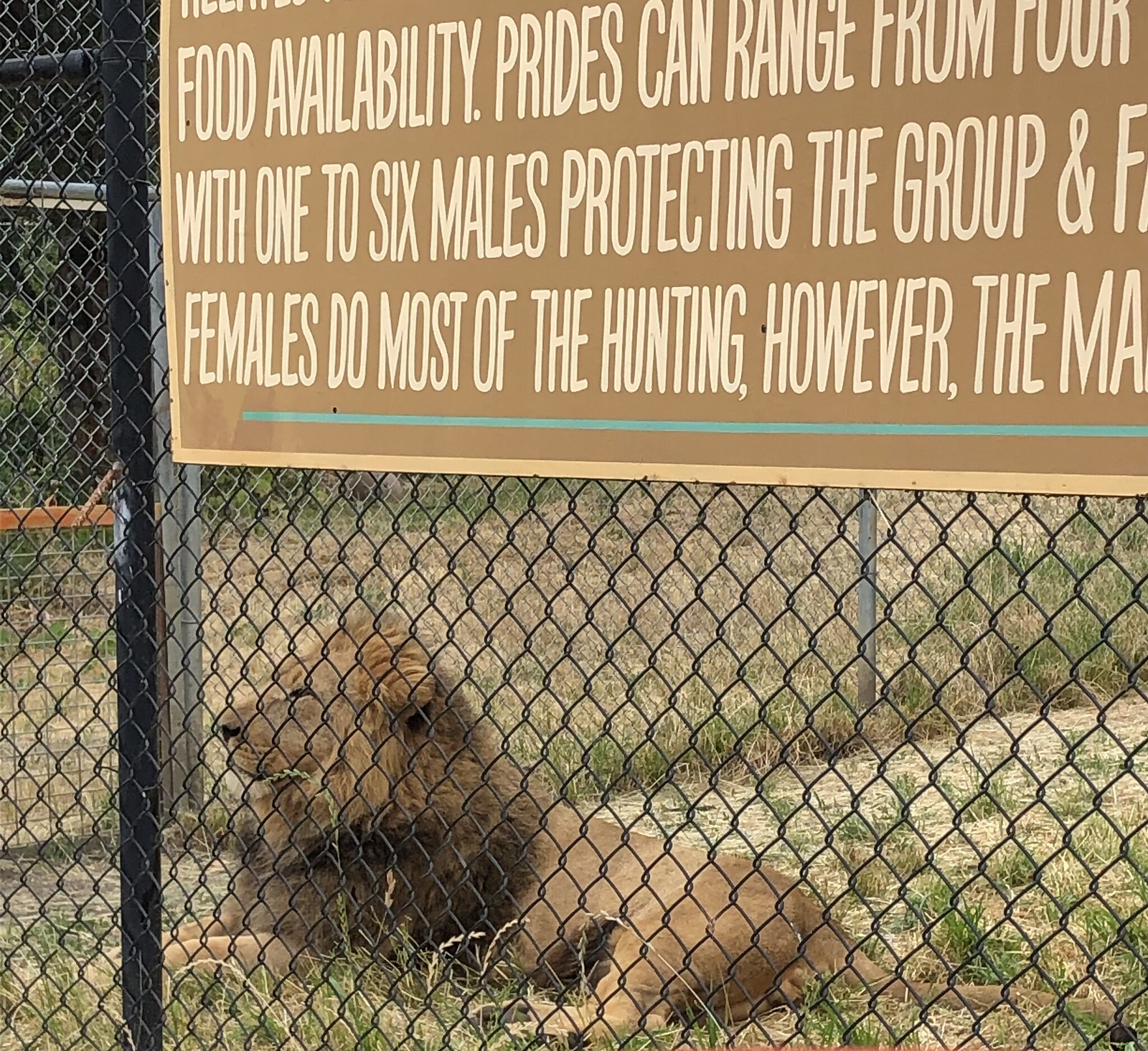A detailed color photograph captures a male lion resting behind a black chain-link fence, likely in a zoo enclosure. The lion, featuring a brown face with a reddish mane and a brownish-tan body, lies on a patch of grass that appears mostly matted and dying, with scattered green patches. A prominent gold sign with white lettering and a green underline hangs on the fence, partly legible, stating, "food availability. Prides can range from four with one to six males protecting the group, and females do most of the hunting, however..." The lion, displaying a somewhat dull expression, looks to the left, its outstretched tail visible against the grassy backdrop. A black pole is also visible in the scene, contributing to the enclosure's structure.